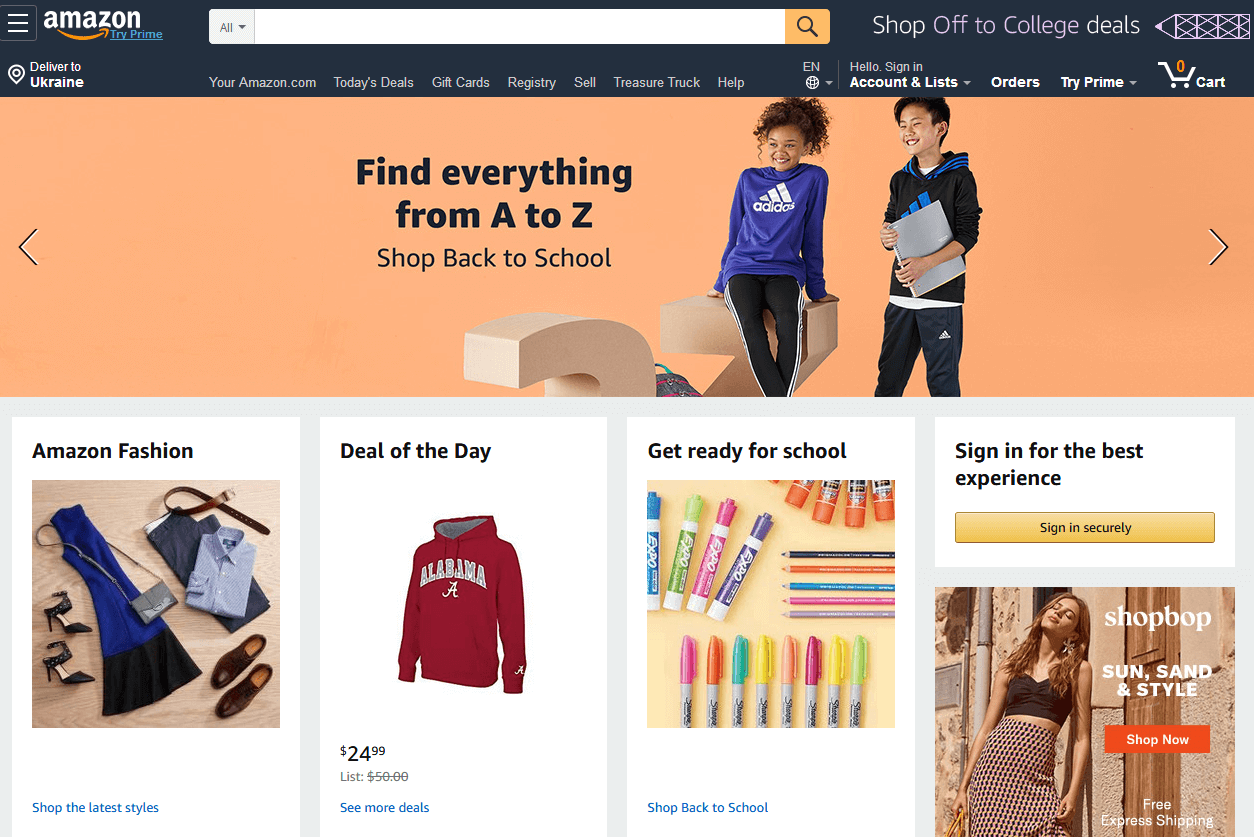**Amazon Home Page Overview**

The Amazon home page features a diverse array of offers and promotions designed to cater to a wide range of customer needs. 

- **Top Section:**
  - **Top Left:** Displays the Amazon Tri-Prime service, now available with delivery to Ukraine.
  - **Top Right:** Promotes special deals tailored for college students with the call-to-action, "Shop Off to College Deals."

- **Promotional Banner:**
  - Set against a vibrant pink background, a prominent banner reads, "Find Everything from A to Z," encouraging users to "Shop Back to School." 

- **Featured Image:**
  - Depicts two children dressed in stylish Adidas outfits, symbolizing the back-to-school season and Amazon's expansive clothing range.

- **Fashion Section:**
  - Below, the Amazon Fashion section showcases a curated selection including:
    - A stylish dress and a matching pocketbook.
    - Men’s trousers, penny loafer shoes, and a belt.
  - A blue hyperlink encourages customers to "Shop the Latest Styles," directing them to the newest fashion arrivals.

- **Deal of the Day:**
  - Highlighted in a white square box, the "Deal of the Day" presents a long-sleeve burgundy sweater with "Alabama" branding, priced at $24.99 (list price $50).

- **Back to School Supplies:**
  - Featuring a box containing essential school supplies like Sharpie markers, glue, and colored pencils with the header "Get Ready for School."

- **Sign-In Prompt:**
  - Finally, a prompt at the bottom encourages users to "Sign in for the Best Experience" to personalize their shopping journey.

This highly detailed layout provides users with clear visual cues and actionable items to enhance their shopping experience on Amazon.